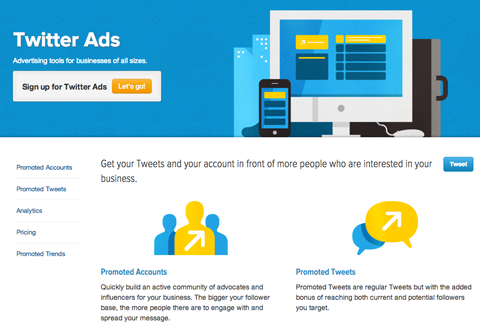At the top of the page is a light brown banner stretching from left to right. On the left side of the banner, white text reads, "Twitter Ads: Advertising tools for businesses of all sizes." Just below this, there is a small white box featuring the text, "Sign up for Twitter Ads," in black. Inside this box is a dark yellow button with the words "Let's Go" written in white.

On the far right of the banner, an animated or clip art image is displayed. This image includes a computer screen, a cell phone, and a briefcase standing on its side. In the far background to the left, there are skyscraper buildings, all rendered in a similar animated style.

Beneath the banner, the background turns white, offering options such as Promoted Accounts, Promoted Tweets, Analysis or Analytics, Pricing, and Promoted Trends. Centrally located is a section that reads: "Get your tweets and your account in front of more people who are interested in your business." Below this message is a blue button labeled "Tweet."

Additionally, more detailed information is provided on the right side of the page. The explanation for Promoted Accounts says, "Quickly build an active community of advocates and influencers for your business. The bigger your follower base, the more people there are to engage with and spread your message." For Promoted Tweets, it states, "Promoted Tweets are regular tweets but with the added bonus of reaching both current and potential followers you target."